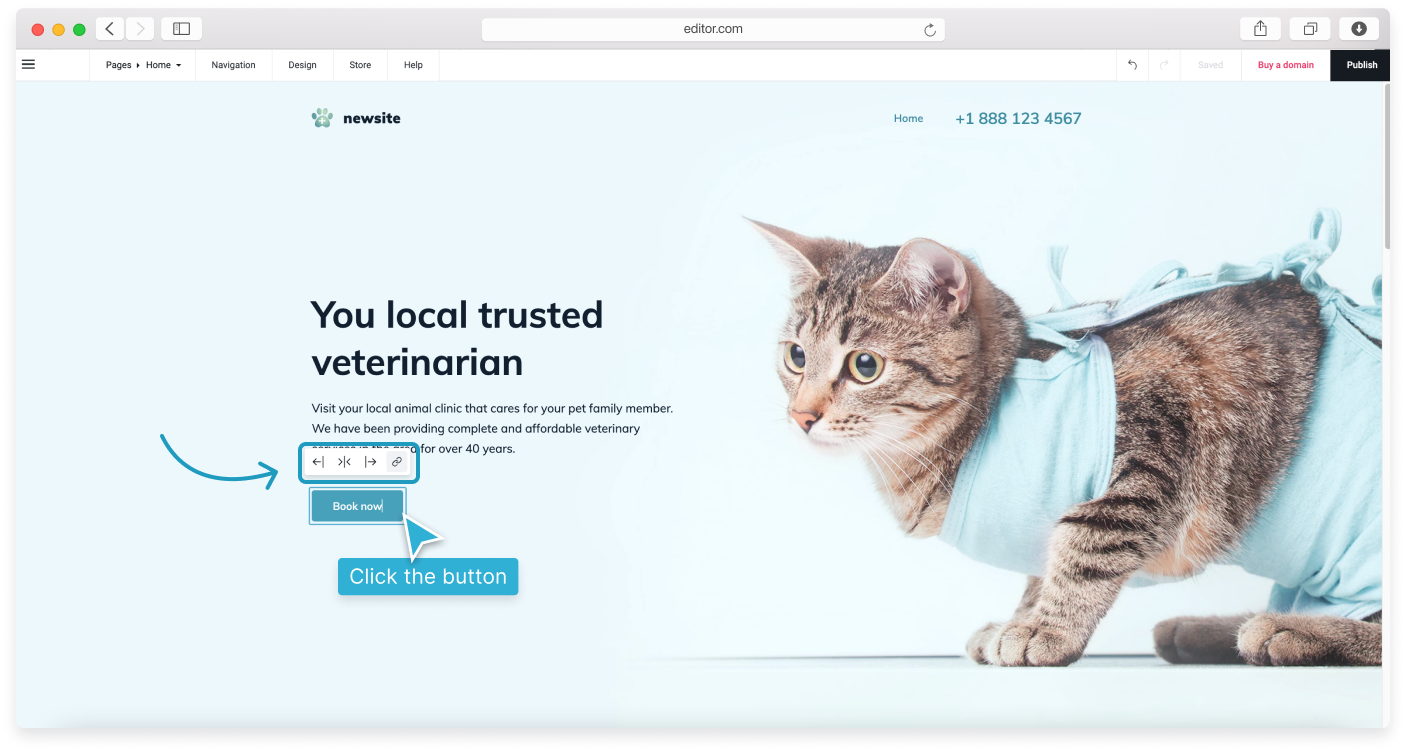This image, captured from a website on a computer screen, features a tiger-striped cat dressed in a light teal protective outfit, possibly indicative of recent surgery or a medical condition. At the top of the image, there's a header with a typo that reads, "You Local Trusted Veterinarian," instead of "Your Local Trusted Veterinarian." Below, a paragraph urges visitors to "visit your local animal clinic that cares for your pet family member," highlighting the clinic's 40-year history of providing complete and affordable veterinary care.

Furthermore, the interface shows that someone has clicked on a "Book Now" button, which is teal with white edging. A detailed layout includes a teal rectangle surrounding navigation buttons and an infinity symbol. Hand-drawn teal arrows are also visible on the screen. The cat’s attire, matching the teal theme, includes the clinic’s phone number and a paw print logo, indicating the newly designed website.